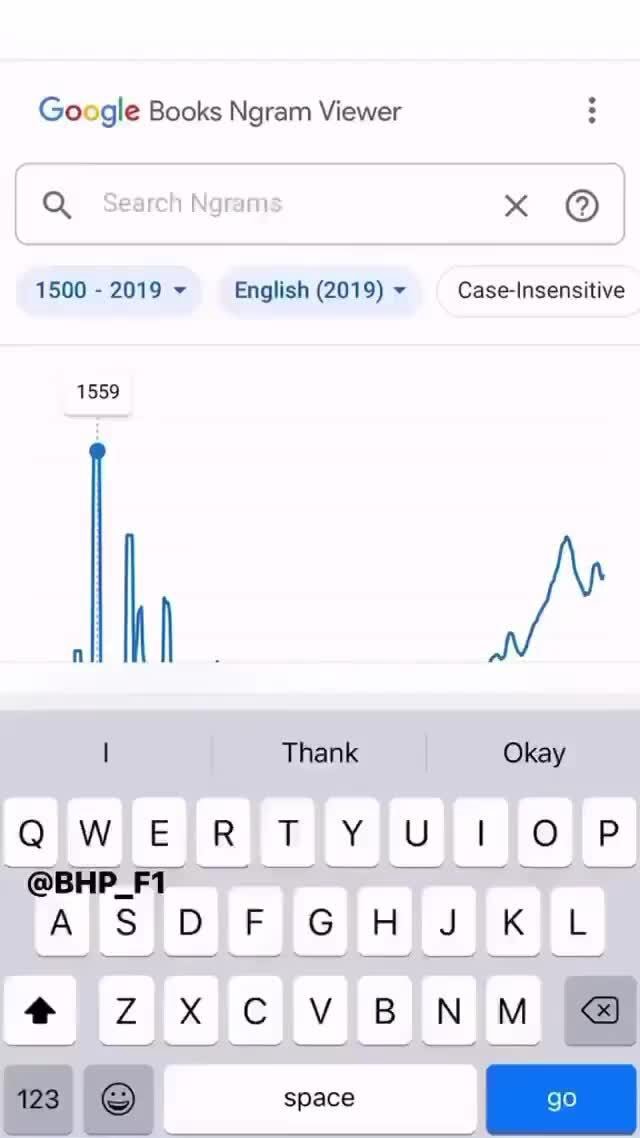The image depicts the Google Books NGRAM Viewer interface. On the top right section, there are three vertically-aligned dots, below which lies a search bar with the placeholder text "search NGRAMS" in gray. The search bar is flanked by a search icon on the left and an 'X' and a question mark icon in a circle on the right. Below the search bar, there are drop-down menus labeled "1500-2019," "English 2019," and an option named "case sensitive." The focus then shifts to a partially visible graph obstructed by a virtual keyboard. The limited part of the graph visible shows a teal line spiking around the year 1559. The virtual keyboard, which has appeared over the graph, features a gray background with white keys and black lettering, and a distinctive blue "Go" button in the bottom right-hand corner. Over the keys 'A' and 'S,' a label reads "@ BHP F1." Additionally, the predictive text area of the keyboard displays the phrase "this is I think okay." The image is filled with various colors including blue, red, yellow, green, black, white, gray, and teal.